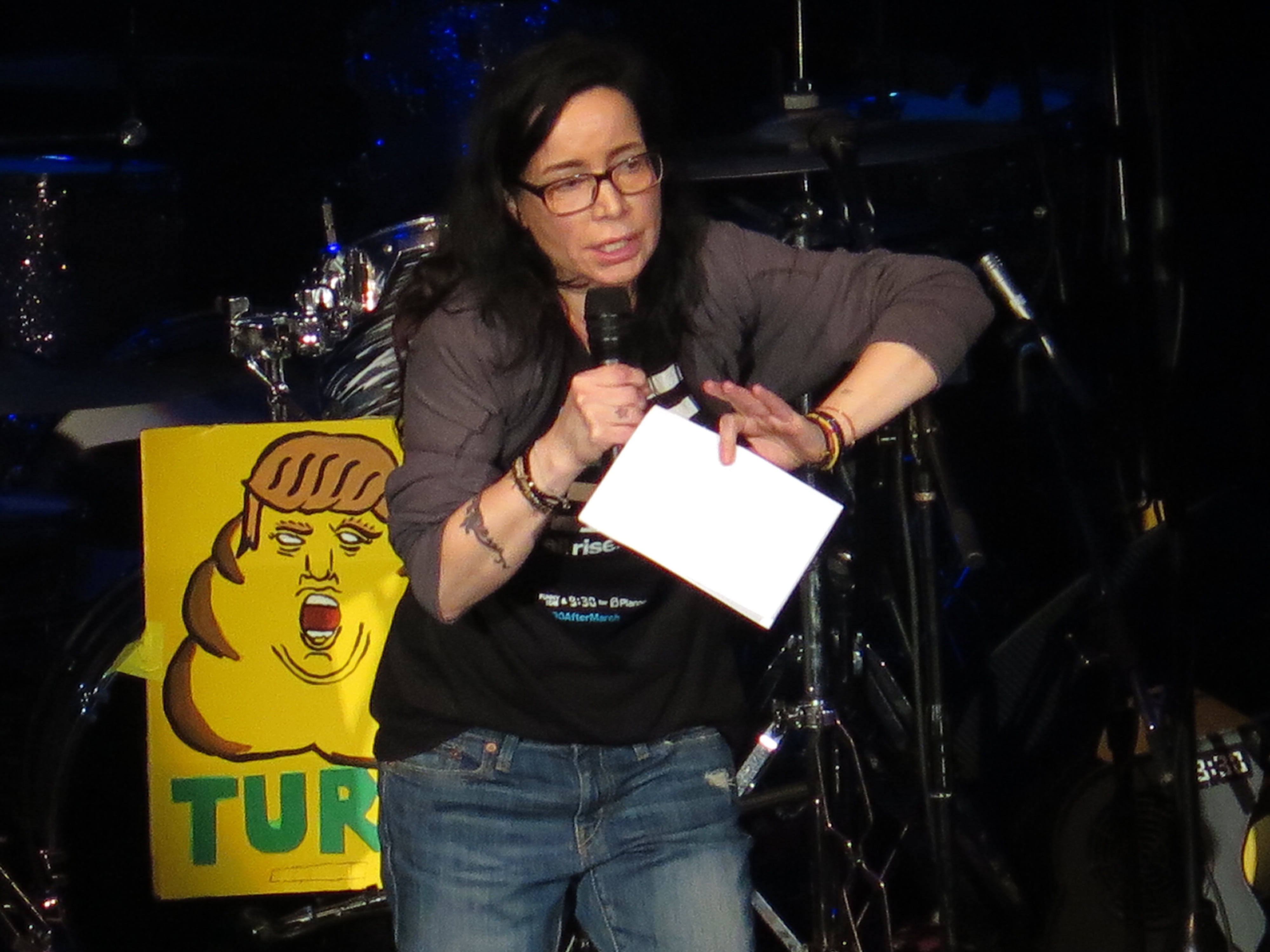The photograph captures a female comedian, likely Janine Garofalo, standing on stage and addressing an audience. She holds a black microphone in her right hand and a piece of white paper in her left. She is dressed in a black t-shirt with unreadable white writing, layered over a long-sleeved gray shirt, and wears blue jeans. Her long brown hair flows down, and she has glasses on her face along with a visible tattoo on her right arm. Behind her is a drum kit with metal cymbals and hi-hats, predominantly black in color. A notable feature in the background is a yellow hand-drawn poster depicting a caricature of Donald Trump as a turd, with green letters partially spelling "T-U-R." The comedian stands central in the image, engaging with the audience in what appears to be a lively performance.